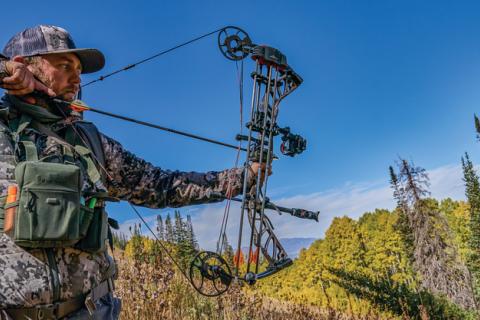The photograph captures a man clothed entirely in camouflage gear, including a cap and a uniform that features shades of grey, light grey, dark grey, or green. He is positioned outdoors, surrounded by a dense forest of trees with some appearing yellow and brown, likely due to seasonal changes. The man is in the action of aiming a sophisticated bow, equipped with mechanical elements such as two wheels at the top and bottom, suggesting a compound bow. This bow is being drawn back as if preparing to shoot. He carries a small dark green olive backpack strapped across his chest. A bright blue sky forms the backdrop, adding clarity and depth to the composition, with distant mountains adorned with numerous trees visible at the bottom of the image.